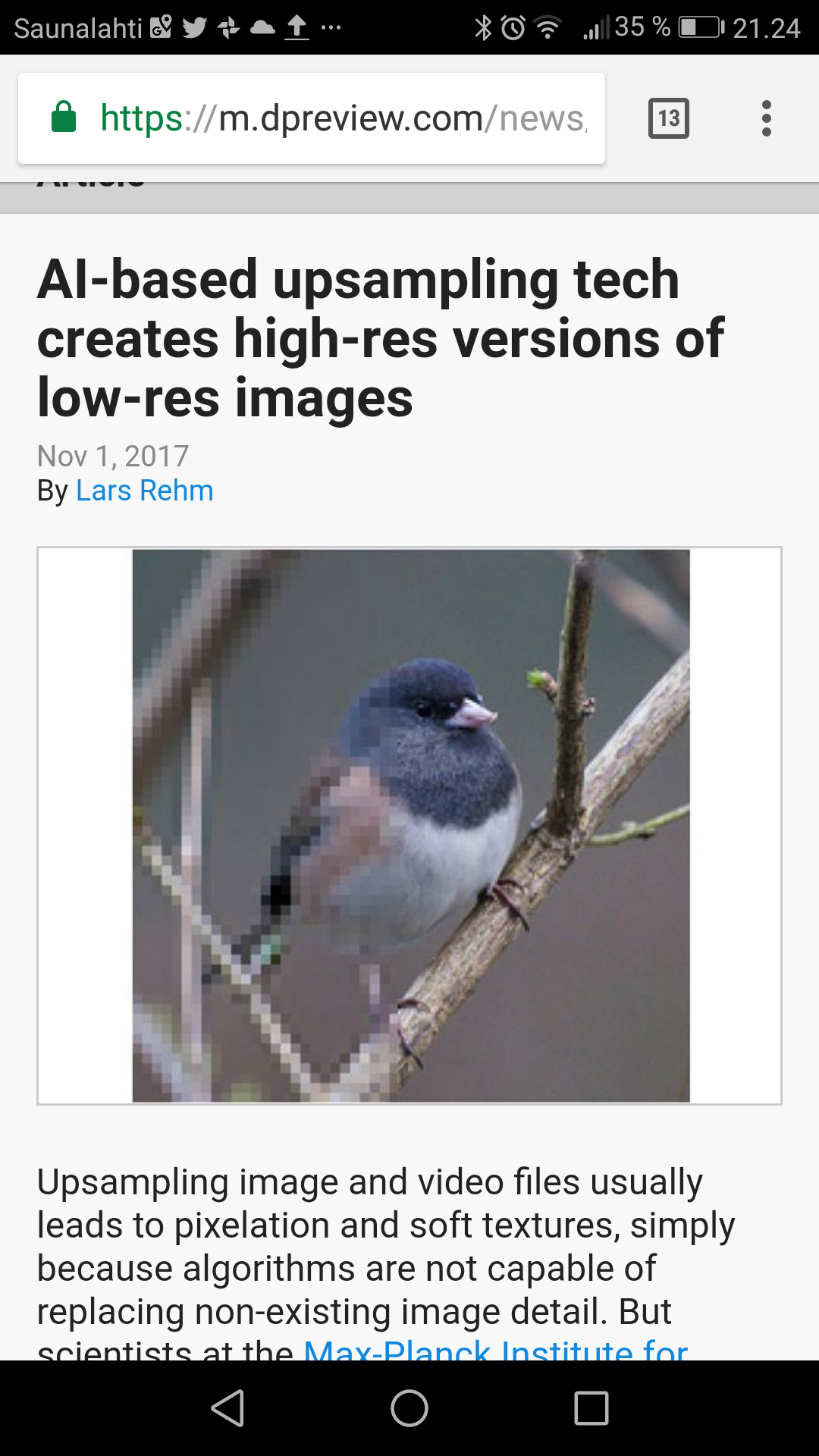This screenshot depicts a web page from a mobile site, with numerous icons and details. In the upper left corner, there are some non-English text and symbols including recognizable icons: the Twitter bird, a pinwheel, a cloud with an arrow pointing upward, and three dots. To the right of these icons, additional symbols are present. The status bar at the top indicates a 35% battery level, Wi-Fi connection, and the time, which reads 21:24.

In the search bar, the URL "https://m.deeppreview.com/news" is displayed, next to a box with the number 13 and another set of three dots. Below the search bar is the title of an article, "AI-based upsampling tech creates high-res versions of low-res images," dated November 1, 2017. The title is in black, followed by the date in gray, and the byline in smaller black text with the author's name "Lars Rehm" in blue, likely indicating a hyperlink.

Under the byline, there is a pixelated image of a bird. The bird has a dark blue head and chest, a white underbelly, and brown wings with some peach coloration, perched on a branch. Beneath the image, text reads: "Upsampling image and video files usually leads to pixelation in soft textures, simply because algorithms are not capable of replacing non-existing image detail." The sentence concludes with a period, but the next line, starting with "But the scientists at the May Plank Institute for," is cut off mid-sentence, with "May Plank Institute for" highlighted in blue, suggesting a hyperlink.

At the bottom of the screenshot, there is a black navigation bar with three icons spaced evenly: a triangle on the left, a circle containing another smaller circle in the middle, and a square to the right.